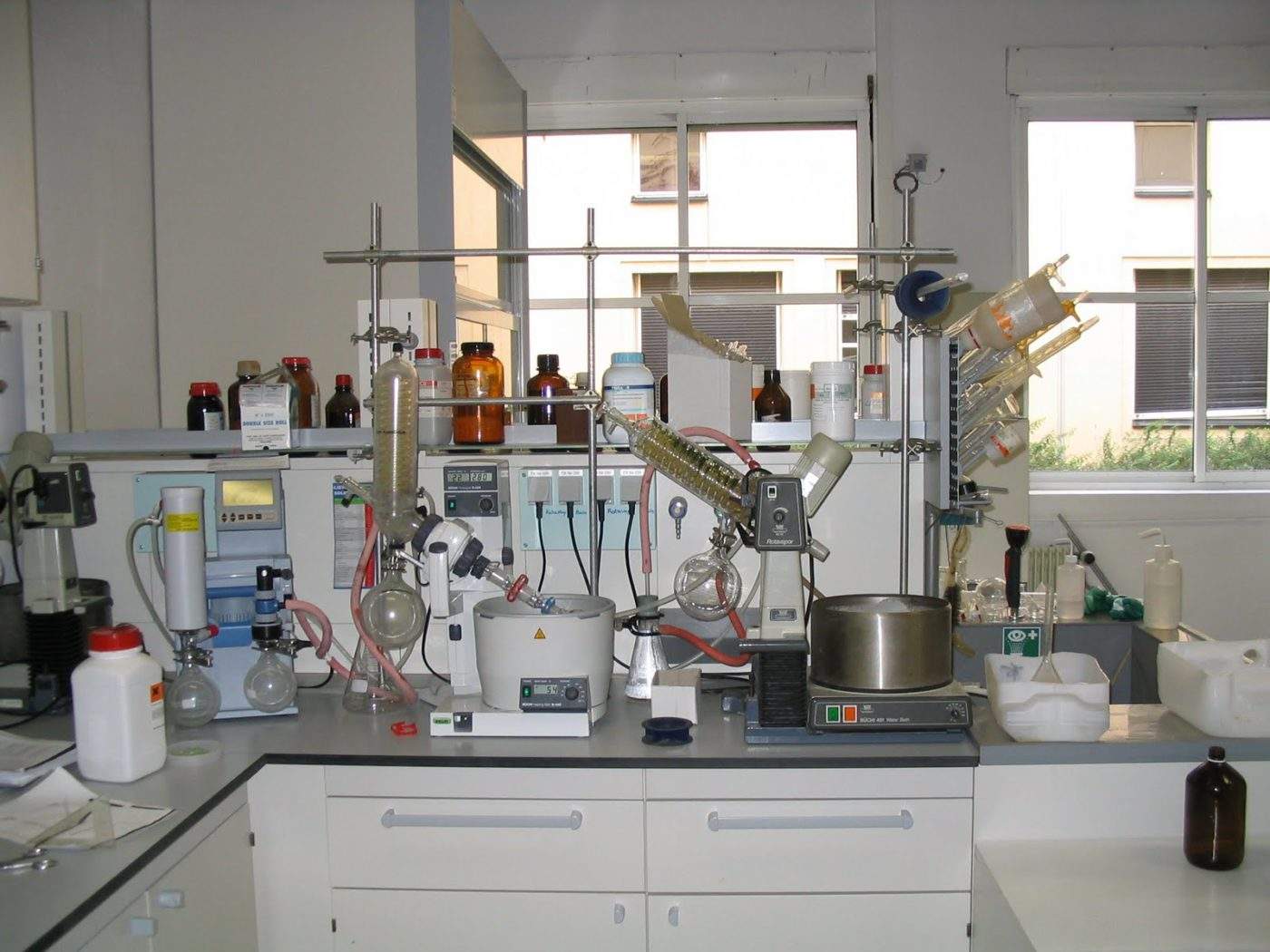The image depicts a corner of a laboratory set up within a home environment, characterized by an L-shaped dark gray countertop surrounded by white drawers and cabinets. The countertop is cluttered with an assortment of laboratory equipment, including various beakers, flasks, and test tubes of different shapes and sizes, as well as multiple brown, orange, clear, and white bottles with lids. Prominently featured among the equipment is a mixer and advanced scientific devices with spinning tubes and machine bases equipped with buttons and knobs, suggesting ongoing chemical or scientific experiments. The backdrop of the image showcases two large, four-pane windows providing a view of a grassy area and another building, adding context to the sterile and commercial-like ambiance of the lab setting. The room's overall appearance is clean and organized, with a bright daytime light filtering through the windows, illuminating the meticulous arrangement of laboratory instruments.